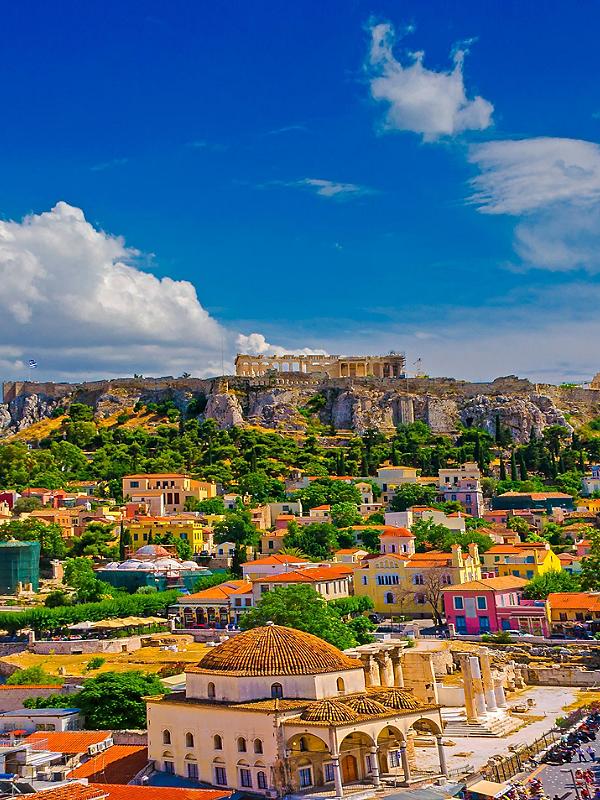The image captures a vibrant, elevated view of a bustling town nestled at the base of a mountain plateau. Dominating the middle ground for a lush expanse of green trees and brightly-colored buildings, the architecture ranges in hues from pinks, oranges, and beige to yellows, blues, and whites, hinting at a style more reminiscent of Indian plaster and clay structures rather than typical American houses. Amidst the eclectic rooftops and colorful facades, a large, cream-colored building with a dark, domed roof stands out prominently in the bottom center of the image, surrounded by verdant greenery. Higher up, the plateau rises majestically, housing what appear to be ancient ruins, adding a touch of historical intrigue to the scene. The sky occupies the top 40% of the photo, a clear blue canvas with a few fluffy, white clouds, enhancing the serene and sunny atmosphere. Sunlight bathes the town, making the vibrant colors pop, and giving the impression that the saturation has been turned up, painting a picture of a peaceful yet vividly dynamic community.